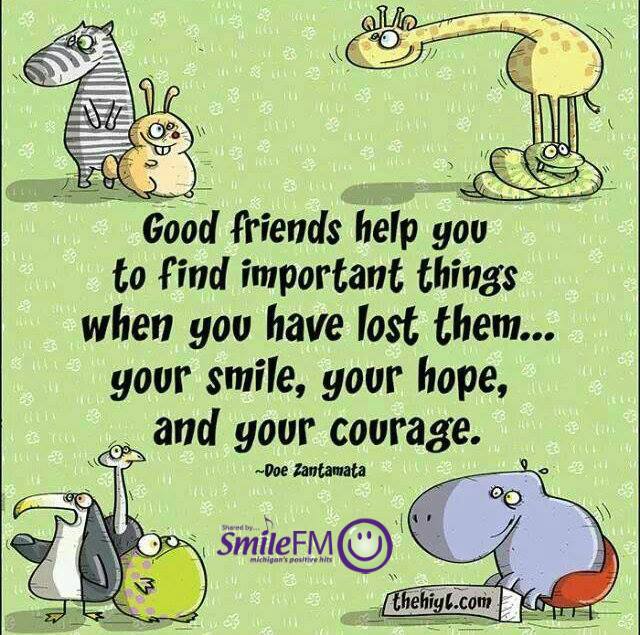The square-shaped poster features a light green background adorned with white squiggly flowers and grass. In each of the four corners, there are cartoon drawings of various animals, seemingly out of a children’s book: a giraffe and a snake in the top right, a rabbit and a zebra in the top left, penguins and a frog in the bottom left, and a hippo holding a sign in the bottom right. In the center of the poster, in black letters, the text reads, “Good friends help you to find important things when you have lost them… your smile, your hope, and your courage. - Doe Zantamata.” Below this, in purple lettering, it says "Smile FM" with the "i" dotted by a musical note and a smile emoji next to it. The hippo’s white sign at the bottom reads "the h-i-y-l dot com."